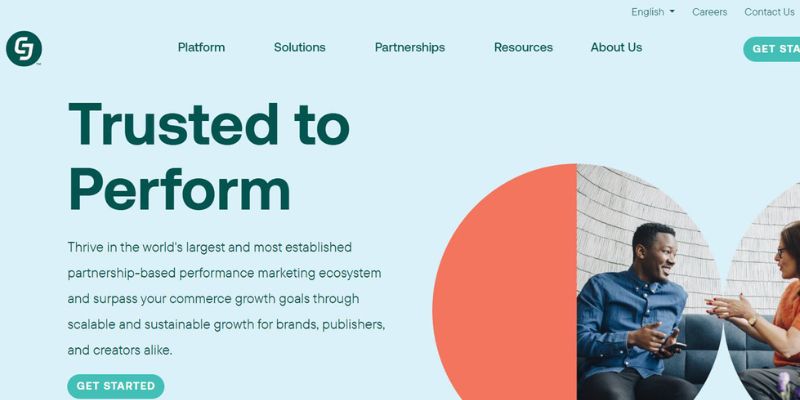The image appears to show a webpage designed to promote "ecosystem commerce growth." In the upper left corner, just below the top left edge, there is a logo consisting of the letters "CJ" in white, encased in a green circle, signifying the company's emblem. Near the top right corner, the word "English" is visible, with a dropdown menu that allows the language to be changed. The top section of the webpage also features links to the "Career" and "Contact Us" sections.

Positioned centrally but slightly to the right of the company logo, there are five clickable options labeled "Platform," "Solutions," "Partnerships," "Resources," and "About Us." Additionally, there is an eye-catching "Get Started" button, characterized by white text set within a green oval, although the word "started" appears to be partially cut off.

Beneath these menu options, the image showcases two spheres and a scene of a man and a woman engaged in conversation while seated on a couch. The man, who is Black with short hair, exudes a cool demeanor, giving a thumbs-up and pointing towards the woman. He is dressed in a buttoned-up dark denim shirt paired with black pants. The woman, adorned in an orange shirt and glasses, is animatedly gesturing with her hands. 

To the left of this interaction, there is a large text in green that reads "Trusted to perform." Below this, a smaller yet prominent text states, "Thrive in the world's largest, most established partnership-based performance marketing ecosystem and surpass your commerce growth goals through a socially sustainable growth path for brands, publishers, creators, and beyond." At the bottom of this section, the phrase "Get Started" is once again displayed, encouraging user engagement.